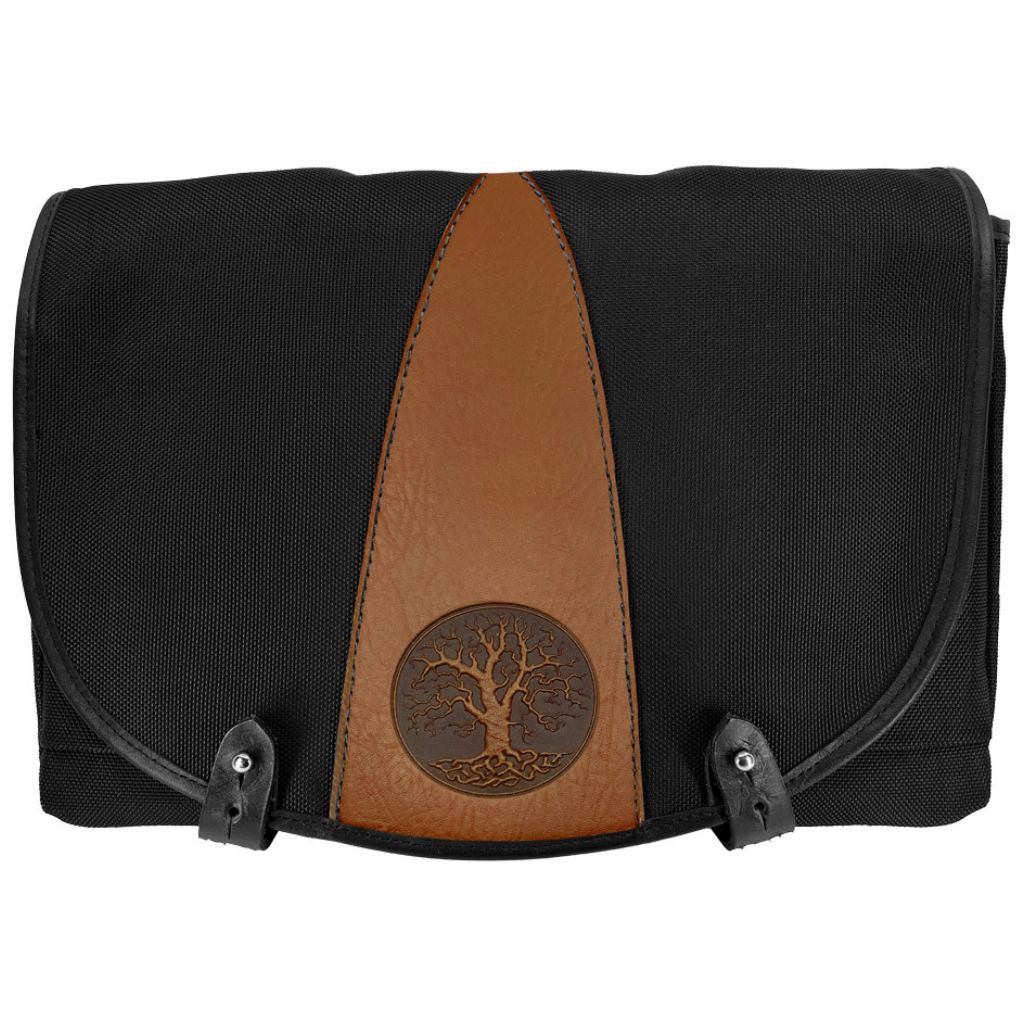This photograph features a satchel or purse-style bag against a white background. The bag has a predominantly black, heavy cloth material, giving it a sturdy appearance. Its body is rectangular with a large, curved flap at the front, which secures with two dark leather clasps on each side, fastened by small silver buttons.

Prominently in the center of the flap is a distinctive tan leather design, highlighted by a black stitched border. This centerpiece displays an elegant, engraved tree motif, depicting detailed roots, a broad trunk, and intricate branches extending in all directions. Below this tree design, the leather area forms an elongated triangle, broad at the bottom and narrowing toward the top. Completing the bag's aesthetic are two small buckles at the bottom, adding a touch of metallic detail to its overall sophisticated look.